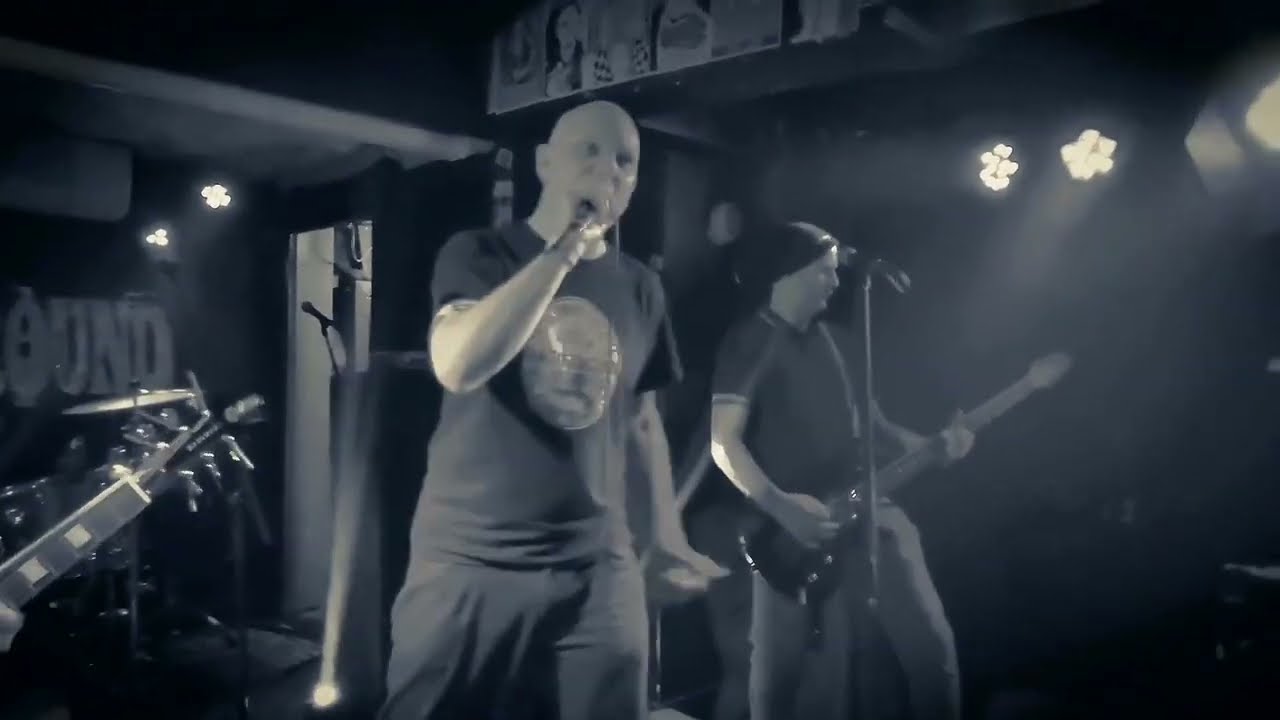This black and white photograph, taken inside a dimly lit and hazy nightclub, captures a dynamic moment of a rock band performance. The central focus is on a bald man holding a microphone, likely singing, dressed in a graphic dark t-shirt and dark pants. He faces slightly to the right, illuminated by some directional lights from the ceiling. To his right stands a guitarist, donning a cap, a dark shirt, and lighter pants, concentrating on his instrument with a microphone stand before him. A portion of another guitar is visible on the far left, indicating another band member just out of frame. The surrounding environment features a couple of bright lights on the rafter and an open doorway in the background. Various posters or signs hang from the ceiling, adding to the atmosphere of the club. The scene is busy yet shadowy, with spotlights creating a stark contrast against the surrounding darkness, capturing the intensity and mood of the live performance.